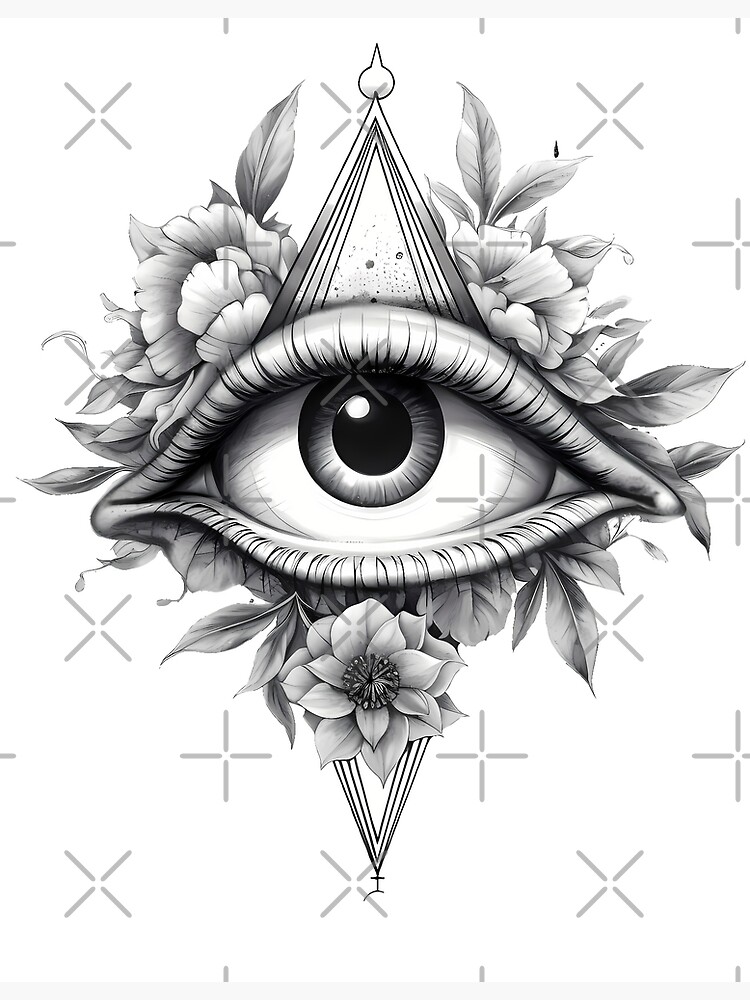The black and white artwork depicts a singular, wide-open eye at its center, surrounded by intricate eyelashes and a detailed eyelid. At both the top and bottom of the eye, triangles are seamlessly integrated into its design. Encircling the eye are numerous meticulously drawn flowers and leaves, including a prominent flower at the bottom featuring several petals. The background is predominantly white with lighter marks forming cross signs and X shapes, which appear to function as watermarks. The overall composition is very detailed and carefully executed, giving the sense that the eye is intensely staring out from the artwork.